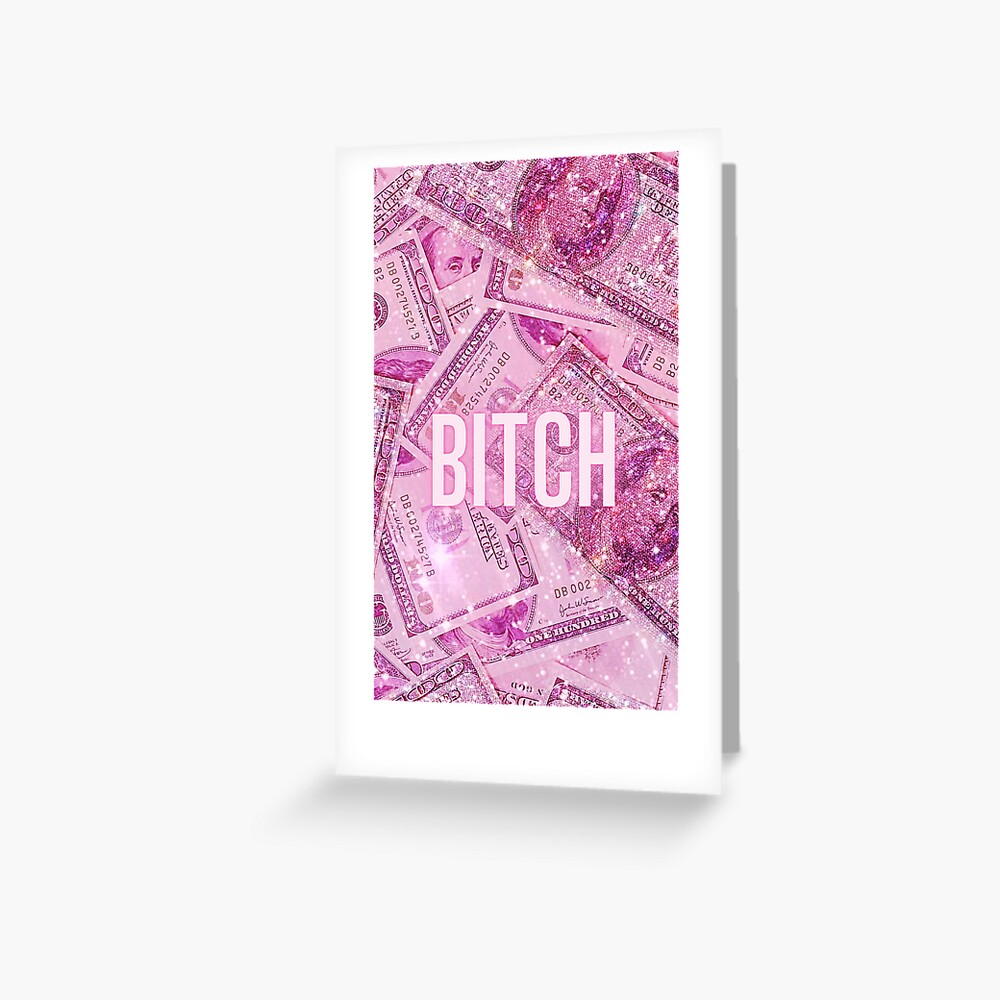The image is of a white-framed artwork hung on a white wall, casting a slight gray shadow to its side. This evocative piece features $100 bills scattered and layered haphazardly, all tinted in a pink or purple hue with a glittery sheen. Dominating the center of the artwork is the word "BITCH" in bold, whitish light pink letters. The visually striking composition of money and provocative text suggests a commentary on wealth and its implications. The frame around the artwork is approximately an inch wide, with the entire assembly presenting a cohesive yet chaotic aesthetic.